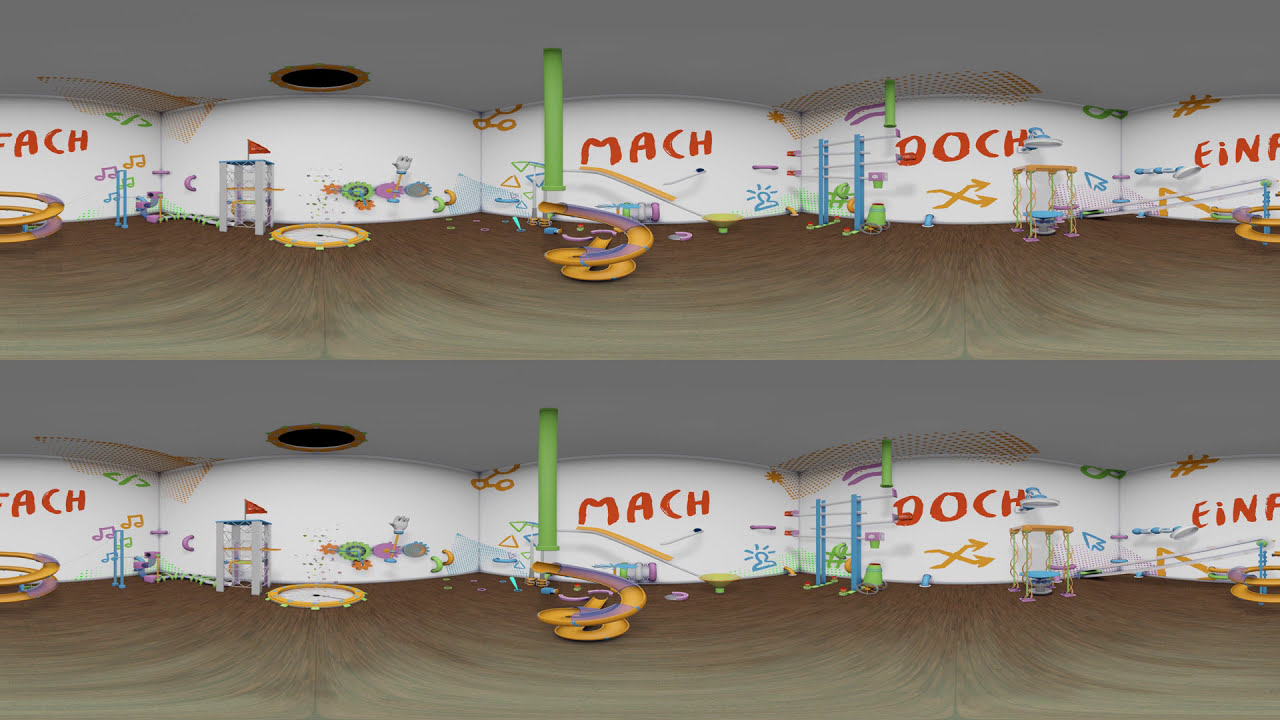This image appears to be a distorted or panoramic cartoon-like depiction, reminiscent of a video game or a child's playground environment. It is notably divided and duplicated, with the top half being an exact replica of the bottom half, resembling the setup of certain VR programs. At the center of the image, a green pipe is suspended in the air, leading to an orange and purple serpentine-shaped slide. The scene features a variety of playful elements arranged across what looks like five sections, each containing different objects such as balls, buckets, cartoonish hands, a mini trampoline, and possibly other toys.

The background consists of white walls adorned with red hand-painted lettering spelling out "FACH," "MACH," "DOCH," and "EIN," though the last letter of the latter word is obscured. Various drawings, including arrows and shapes in orange and blue, also decorate the walls. The flooring is described as having a swirled wood grain pattern, and the ceiling, which is darker gray, features a notable black hole with a gold ring around it. Blue stable shelves are visible on the side, contributing to the eclectic array of trinkets and objects that give the room a whimsical and child-friendly atmosphere.